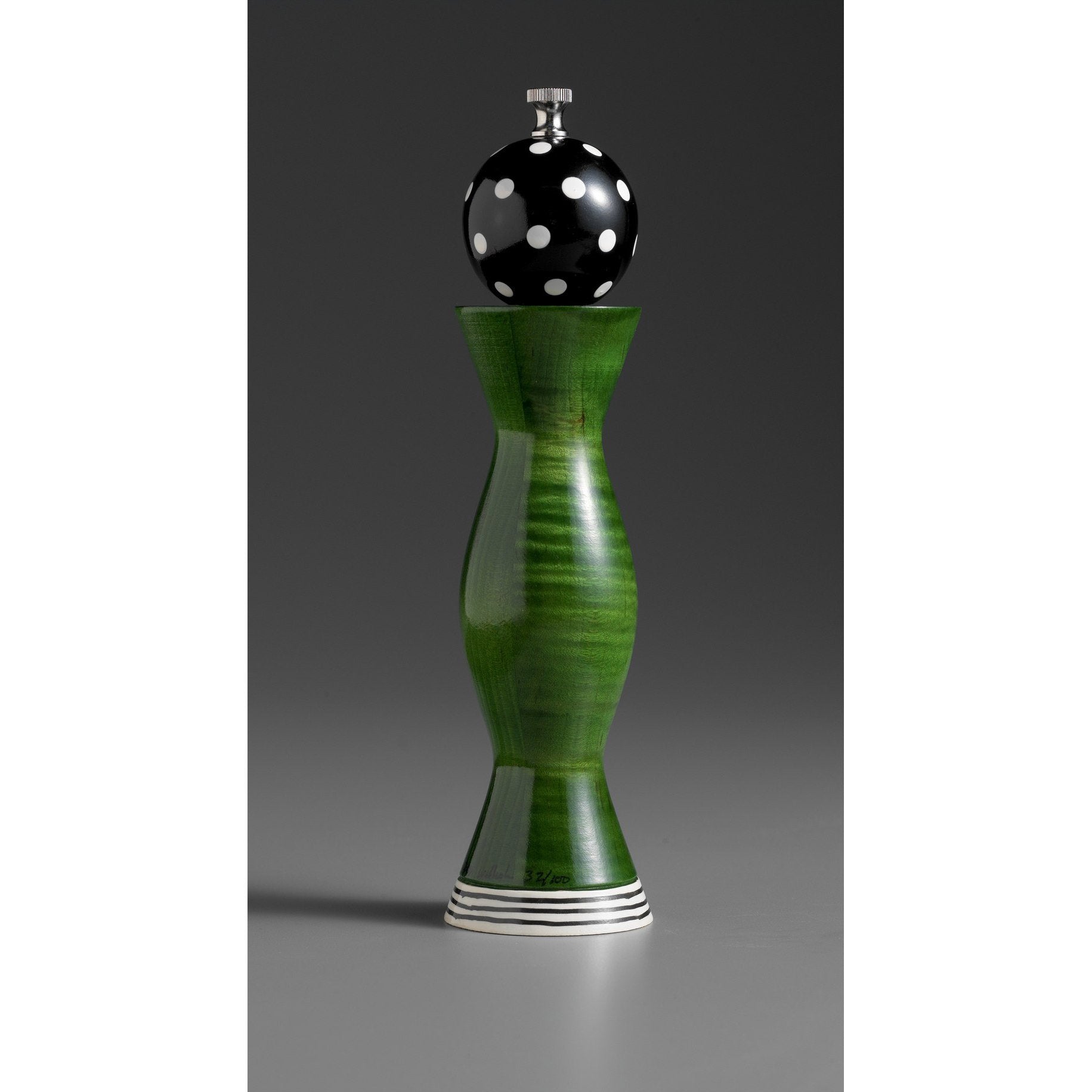In the image, there appears to be an intriguing object that is difficult to classify definitively. The object features a circular top that is decorated with a black background and white polka dots. Emerging from this circle is a metal screw, suggesting a functional component often found in lamps but not exclusively so. 

Below the circular top, there is a curvaceous green platform that resembles the silhouette of an hourglass or an elegant, shapely woman. This platform bows outward, curves inward, and then bows outward again before tapering towards the bottom in a fishtail-like shape.

At the base, the object is adorned with alternating white and black stripes. Given the combination of these elements, it is unclear whether the object is a vase, a component of a lamp, or an abstract decorative piece.